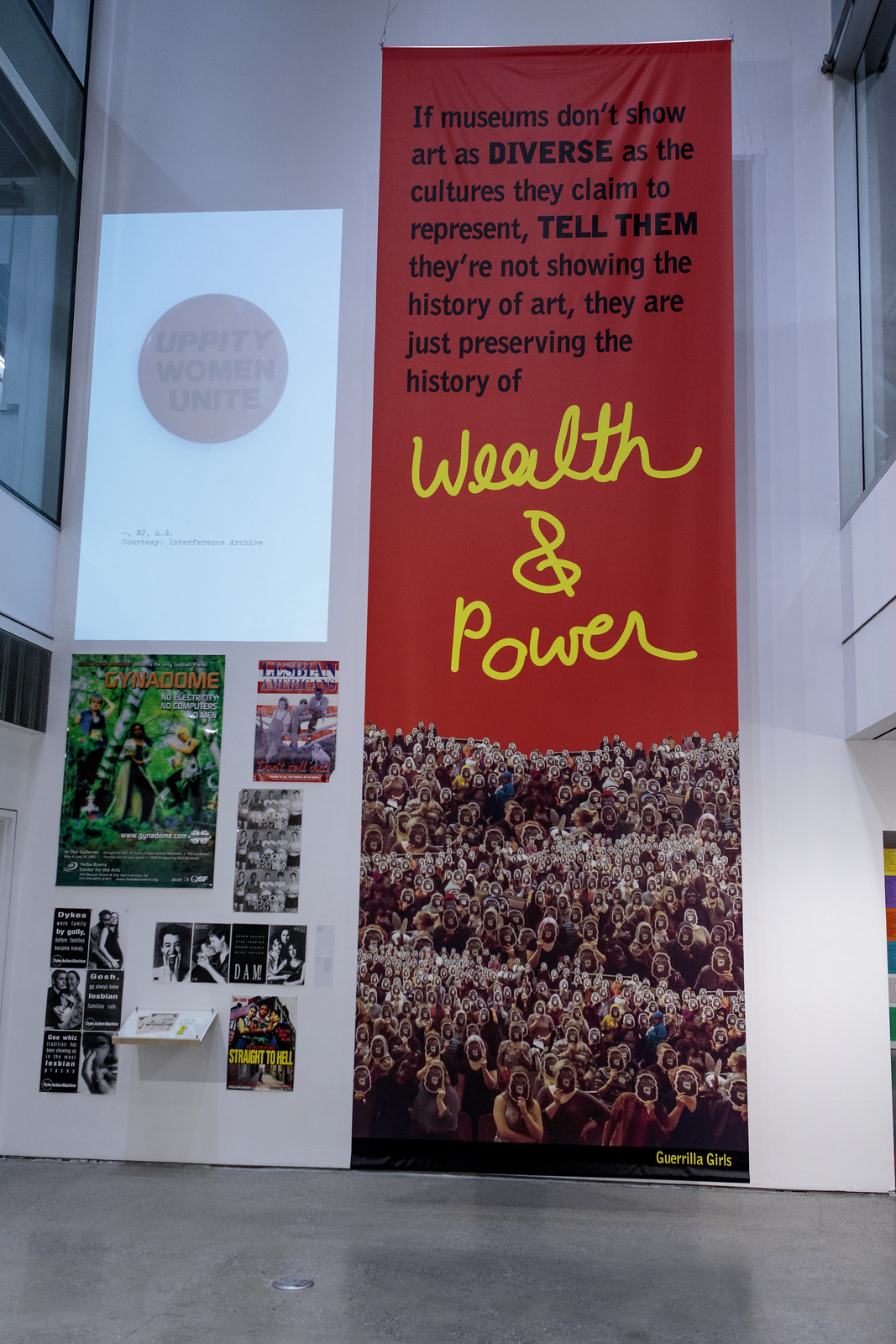In this photograph, the primary focus is a large vertical banner occupying the center of a predominantly white wall, with narrow glimpses of adjacent walls on either side, each featuring windows. Below, shiny gray concrete or linoleum flooring reflects the light. The upper three-fifths of the banner is red, inscribed with the message in bold black print: "If museums don't show art as diverse as the cultures they claim to represent, tell them they're not showing the history of art, they're just preserving the history of wealth and power." The phrase "wealth and power" stands out in large yellow cursive. Beneath this text is an aerial photograph displaying a dense crowd of indistinct people.

To the left of the banner, the wall is adorned with various smaller posters. At the top, a prominent poster features a white background with a gray circle and the phrase "Uppity Women Unite." Below this central poster, there is a collection of smaller, colorful posters in various shapes, including green, red, black, and white designs. The overall scene suggests an art gallery or cultural space, possibly at an entrance, given the modern architectural elements and the window visible to the upper left.